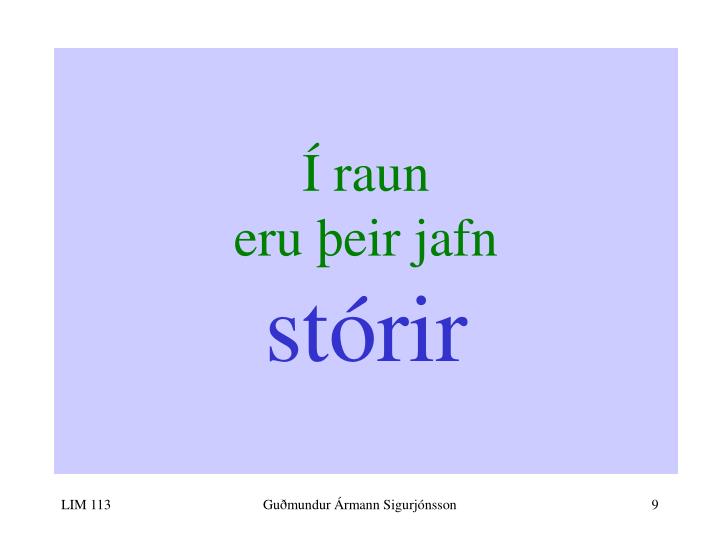The image, resembling a slide from a slideshow, features a central, light purple (lilac) rectangle with a white border. The background is consistently shaded in light blue, almost gray. Prominently placed on the lilac block, in uppercase green text, is a sequence that begins with a capital "I" accented with a small acute line. Following this are the letters "R-A-U-N-E-R-U-P," then on subsequent lines, "E-R-U" and "P-E-I-R," ending with "J-A-F-N." Below this, in larger, dark purple text, is "S-T-O" accented with an acute mark, followed by "R-I-R." Near the bottom of the image, in small black text on the white border, are the details "L-I-M-1-3-T-E-N-G," along with names "G-U-D-M-U-N-D-U-R," "A-R-M-A-N-N," and "S-I-G-U-R-J-O-N-S-S-O-N," concluding with the number "9."